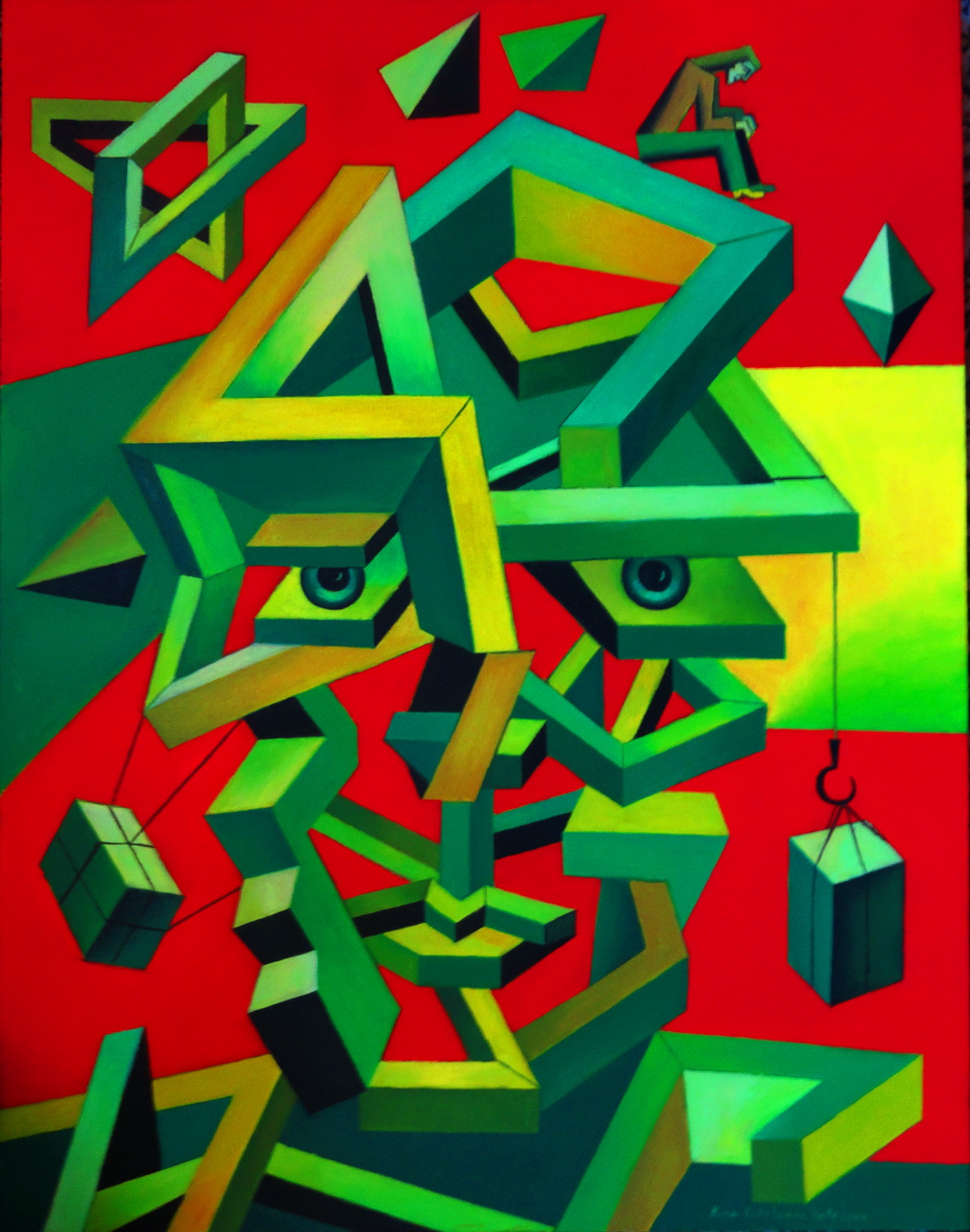This vibrant painting, rooted in abstract art, presents a fascinating composition of geometric shapes that collectively form a robot-like head. The background is a rich mix of blocky red tones interspersed with shades of lime green, dark green, medium green, yellow, and occasional neon highlights. Dominating the mid-right of the canvas is a large, neon green square, partially obscured, while parallel on the mid-left, a dark green triangle or potentially a covered rectangle balances the scene.

Central to the image is the robot’s face, a complex assembly of three-dimensional shapes. Two round eyes in a dark emerald green appear amidst varied rectangular shapes in dark green, light green, and yellow hues. These shapes, both open and interconnected, mimic facial features: a rectangular structure suggests the nose, a gear at the bottom middle symbolizes lips, and additional rectangles imply the chin and hair. Horizontal, curved rectangular shapes hint at the robot’s neck and body, with small boxes or gifts hanging on hooks and strings akin to earrings.

Above, a range of cube and pyramid shapes scatter across the composition, with a tiny figure perched thoughtfully on the top right of the robot's head. This figure, dressed in a brown shirt and green pants, gazes downward, enhancing the contemplative atmosphere of the piece. The painting, with its vivid colors and intricate details, may symbolize the workings of a mind through its mechanical and humanoid elements.